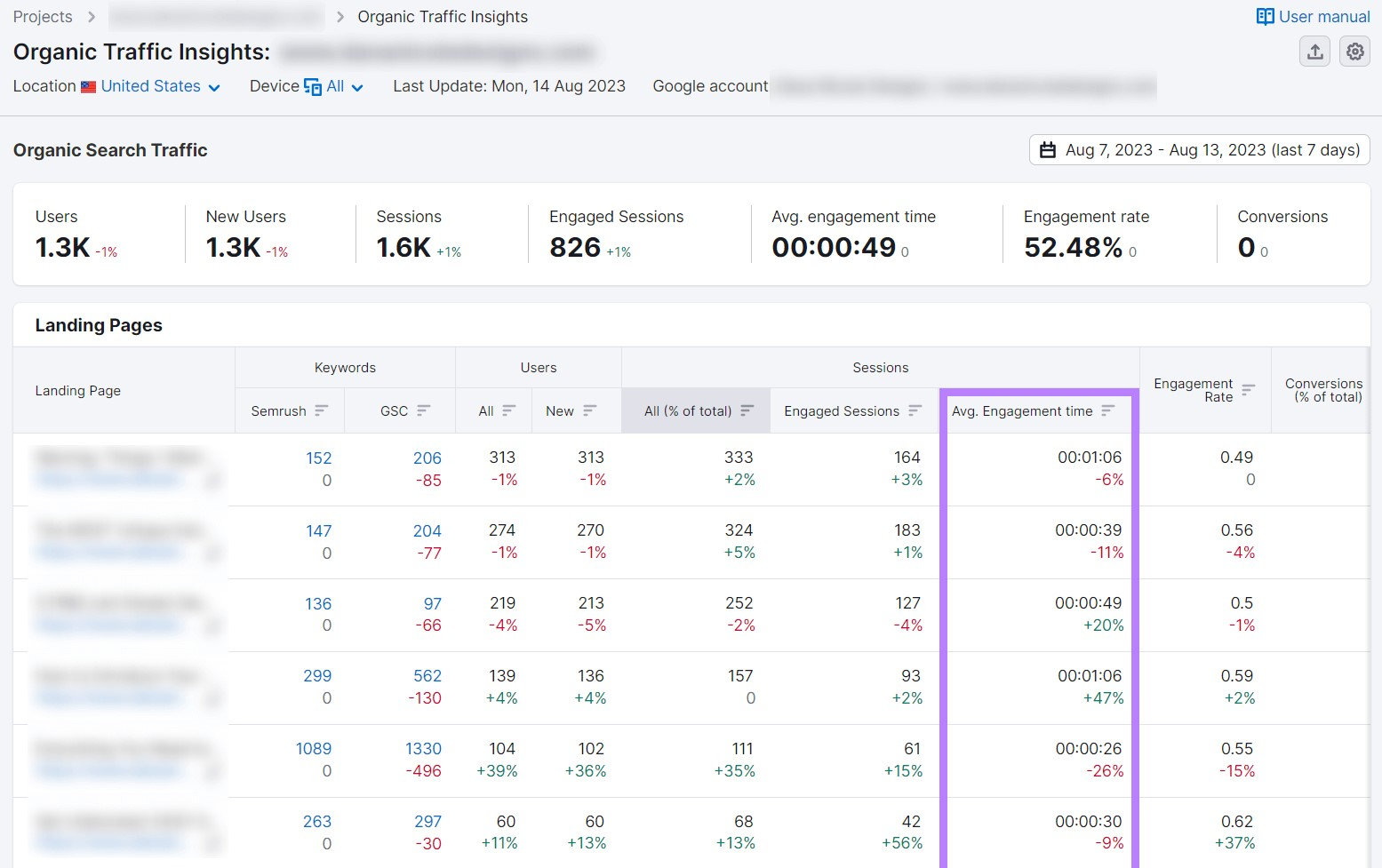Screenshot of a dashboard interface displaying a hierarchical list and organic traffic insights metrics. On the top left, the screen reads "User Manual" accompanied by an icon resembling a manual. Directly below appears a hierarchical list starting with "Projects," followed by a blurred segment, and then an arrow pointing to "Organic Traffic Insights."

Within the left sidebar, "Organic Traffic Insights" appears again, followed by additional blurred content. The main section details metrics with the site's location set to "United States" and devices covering "All." There are various user drop-down options available. The last data update is marked as "Monday, 14 August 2023" tied to a Google account.

The core of the dashboard displays a detailed table under the title "Organic Search Traffic," listing various statistics: users, new users, sessions, engaged sessions, average engagement time, engagement rate, and conversions. Numerical values provided include: 1.3K, 1.3K, 1.6K, and 826 for the top metrics. 

Below, repeated engagement figures show a consistent 1.9K across several consecutive rows, highlighting steady or recurring data points.